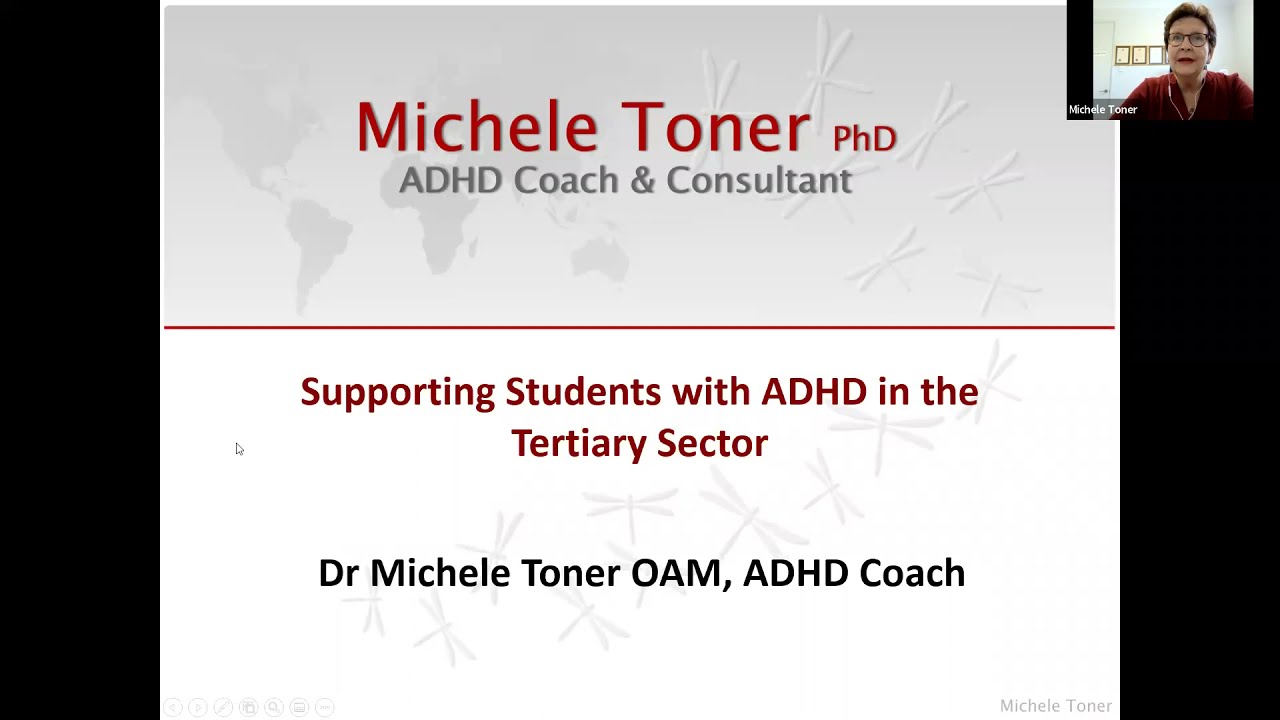This screenshot from a Zoom call captures a presentation by Dr. Michelle Toner, Ph.D., an ADHD coach and consultant. In the upper right corner, a small video window shows Dr. Toner, a woman with short brown hair, wearing black glasses, wired earbuds, earrings, and a red blouse. Behind her, the white wall displays numerous certificates. The main slide prominently features her name, "Michelle Toner, Ph.D.," in red, with "ADHD Coach and Consultant" in gray. The slide title, "Supporting Students with ADHD in the Tertiary Sector," is displayed against a faint world map adorned with dragonfly illustrations. The text, presented in red, gray, and black, reiterates her credentials and name multiple times, emphasizing her expertise and the focus of the presentation.